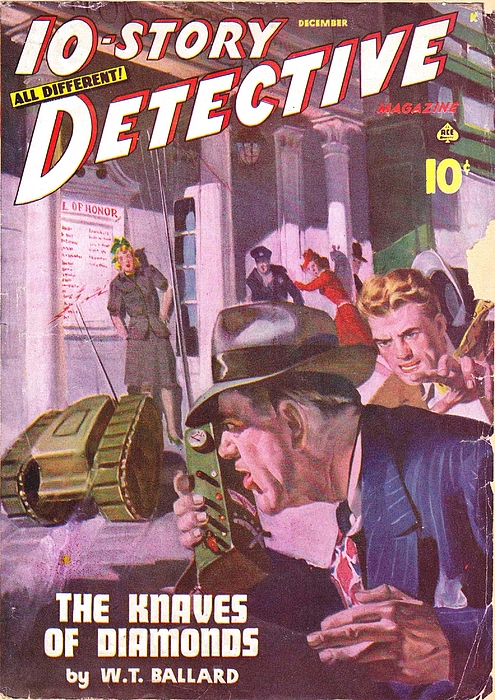This vintage comic book, titled "The Knaves of Diamonds" by W.T. Ballard, is a December issue from Ace Comics, priced at 10 cents. The cover prominently features a character reminiscent of Dick Tracy, decked out in a distinctive navy blue and white pinstripe suit with a walkie-talkie in hand and his iconic hat. In the background, a woman, seemingly clad in a military uniform, stands near a building labeled "Hall of Honor." Beside her is a navy man, adding to the scene's air of intrigue.

Additionally, the cover depicts a woman in a striking red dress and a blonde-haired man in a tan suit, both seemingly in pursuit of the Dick Tracy-like figure. A small, military-style tank with a noticeable antenna and red radio waves radiating from it—a clear nod to the era's depiction of radio-controlled technology—further enhances the drama and action of the scene. This comic book promises an engaging collection of ten unique detective stories, providing a thrilling escape into a world of mystery and adventure.